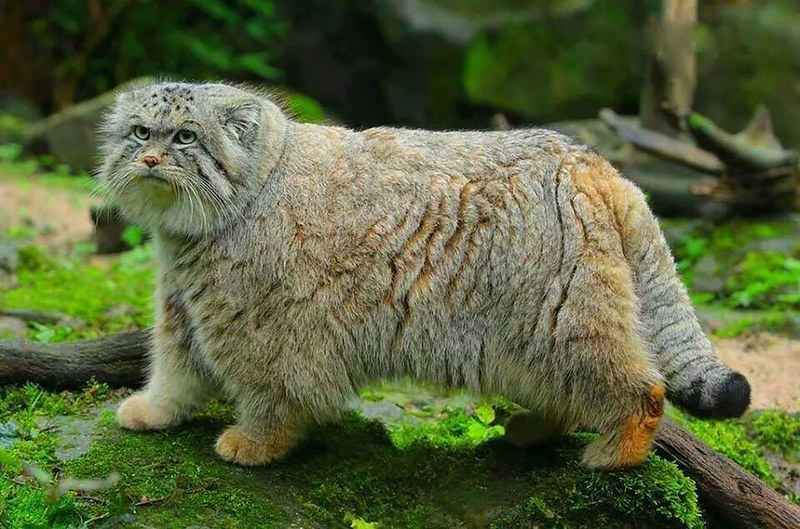This photo, taken in a mossy forest area, showcases a remarkably furry feline that resembles both a house cat and a prehistoric wild cat. The animal, with its exceedingly thick and long fur, gives the impression of being heavily set. It has short ears and a bit of black spotting on its forehead, while the rest of its body is primarily gray with some brown accents. Its fur drapes down almost to its feet, and it possesses a long, fluffy tail with distinct black markings on the tip. The cat’s head features a dense mane of fluff, somewhat reminiscent of a lion. The feline appears to be navigating a forest floor covered in green moss, surrounded by fallen branches, logs, and brown tree trunks, some of which are partially visible among the dense foliage and large moss-covered stones in the background. This image could depict a wild feline species native to an Asian or jungle environment, and the setting evokes a natural, untamed habitat.